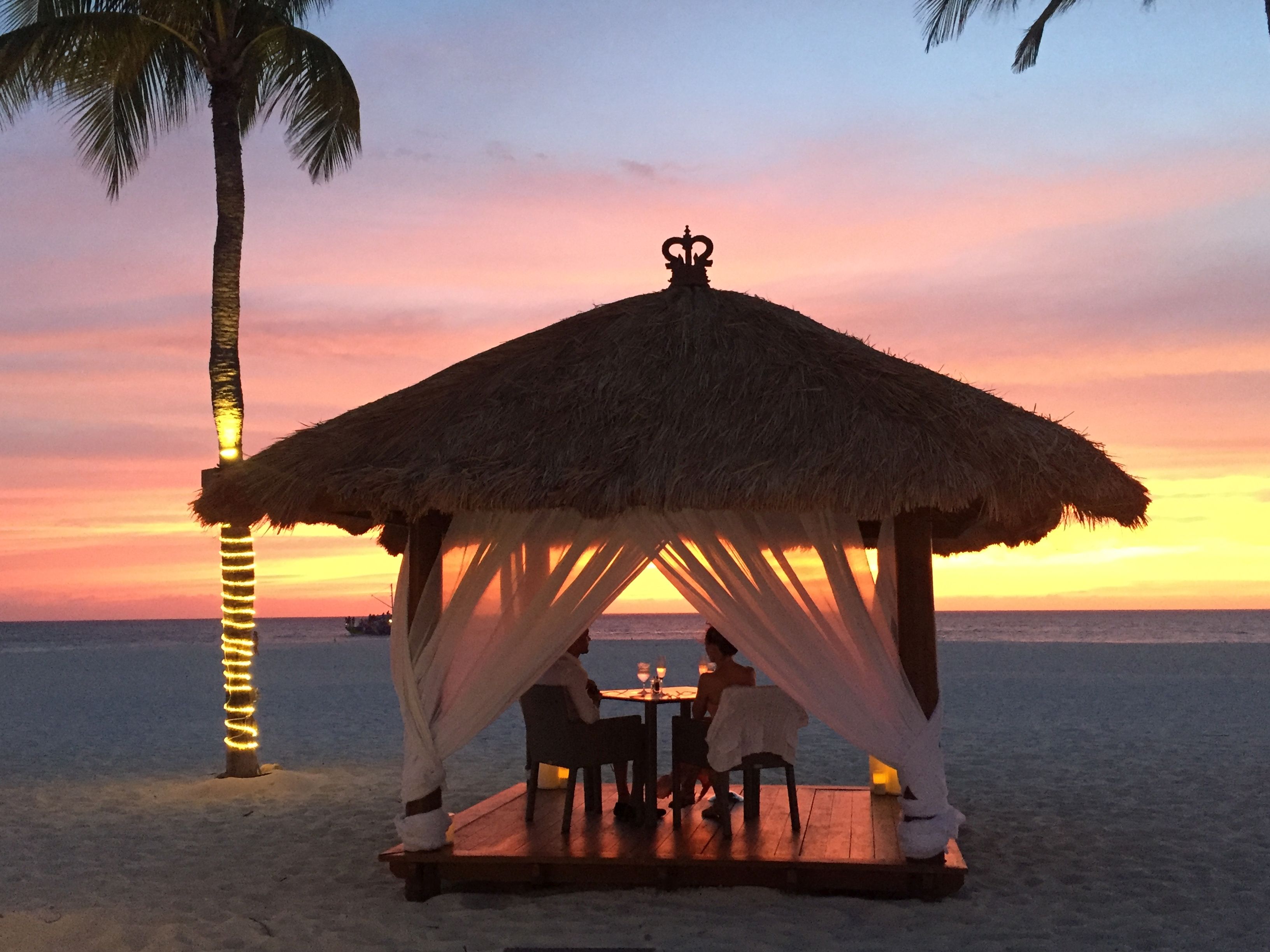A romantic evening unfolds on a white sandy beach as a couple enjoys a serene sunset under a charming cabana. The small wooden platform with a thatched roof is adorned with flowing white sheer fabric wrapped around the visible posts, creating a dreamy ambiance. The couple, seated at a table with two wine glasses, gazes out at the tranquil ocean as vibrant hues of light blue, lavender, pink, peach, and yellow paint the sky. A palm tree on the left, decorated with twinkling lights around its trunk, adds to the enchanting scene, while another palm tree’s fronds peek into the frame from the top right. In the background, the faint silhouette of a boat drifts on the horizon, enhancing the setting’s picturesque and peaceful nature.